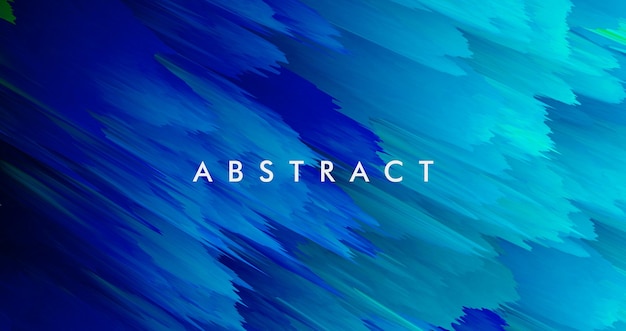This illustration predominantly features various shades of blue, ranging from dark blue on the left, transitioning to medium blue in the center, and culminating in light blue on the right. The artwork is characterized by distinct paint strokes, which mirror this gradient transition – dark blue strokes on the left, medium blue in the middle, and light blue on the right. In the center of the image, bold uppercase white lettering spells out "ABSTRACT," indicating the nature of the art. Additionally, the lower section has more dark blue tones towards the right. A subtle yet striking detail is a thin stroke of lime green situated in the upper right corner, adding a contrasting element to the predominantly blue palette.